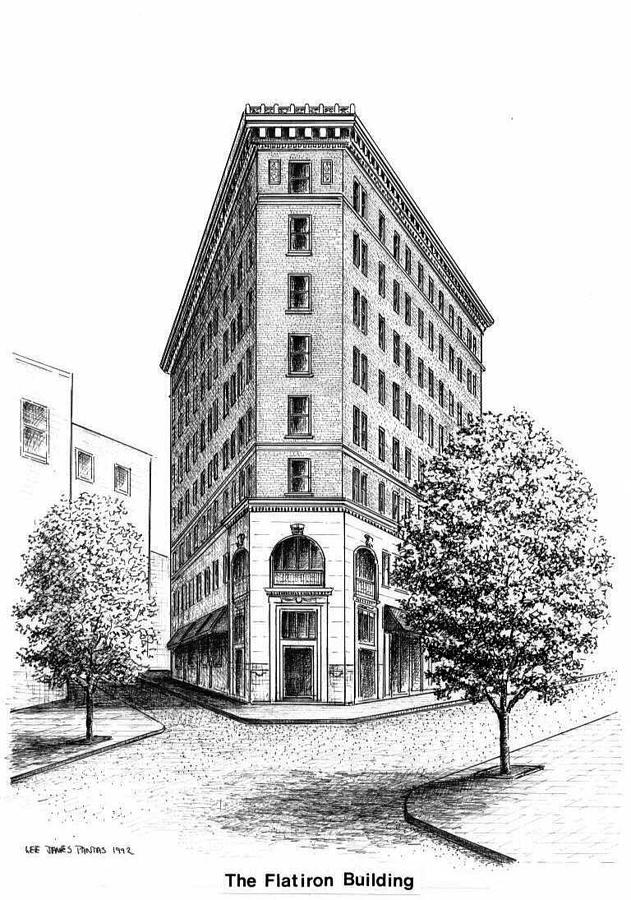This detailed black and white illustration depicts the iconic Flatiron Building in New York City. The building is situated at an intersection where three streets meet, forming a triangular shape, reminiscent of an inverted 'V.' The front of the building showcases six stories above a grand archway entrance, framed by white stones. The arch includes a doorway topped with an awning. On either side of the building, streets lined with trees highlight the urban setting. To the left, two smaller, simpler buildings are visible: a two-story rectangular structure with two windows on the second floor and another building with a single window on the second floor. The sky in the illustration is left white, and shadows loosely outline the trees on the street. The title “Flatiron Building” is inscribed at the bottom of the illustration along with the artist’s credit, “Lee S. James S. Plasters, 1992.”